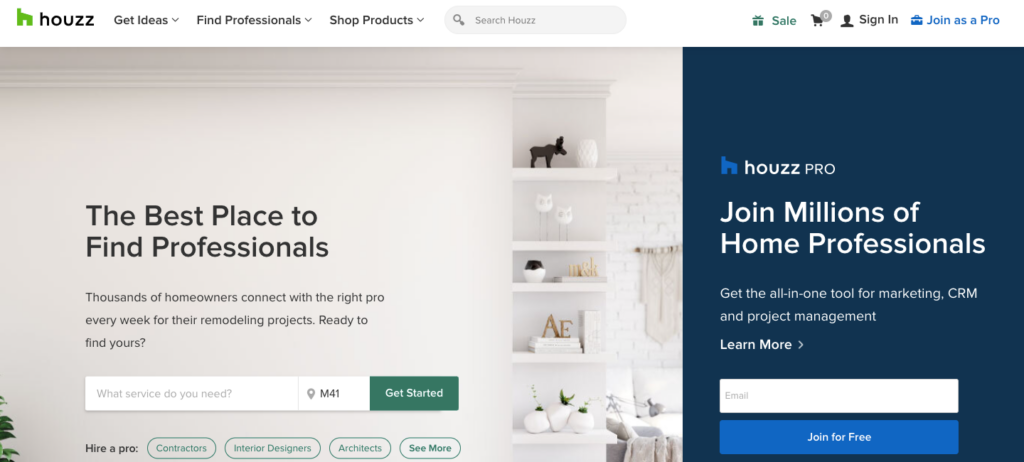The screenshot captures a segment of a professional home improvement website. At the top, the website features a clean, white background adorned with black text and a green logo resembling a house or the letter "H". Adjacent to this logo is the site name "Houzz" in bold letters. The navigation bar includes drop-down menus labeled "Get Ideas," "Find Professionals," and "Shop Products". To the right of these options, there is a search bar followed by links for "Sale," "Cart," "Sign In," and "Join as a Pro."

Beneath the navigation bar, the left-hand section showcases a color photograph of a white wall fitted with white shelves. Superimposed on this image is the text: "The best place to find professionals. Thousands of homeowners connect with the right pro every week for their remodeling projects. Ready to find yours?" Below this, a horizontal bar prompts users to select the services they need with the call-to-action button, "Get Started."

Further down, the text encourages users to "Hire a Pro," detailing potential professionals such as contractors, interior designers, and architects, with associated buttons for each category and a "See More" option.

On the right side, against a black background, features a blue variant of the house logo accompanied by the text "Houzz Pro," inviting users to "Join millions of home professionals" in white font. Additional text in a smaller white font describes the benefits: "Get the all-in-one tools for marketing, CRM, and project management." The section concludes with a prompt for email entry and a "Join for Free" button.